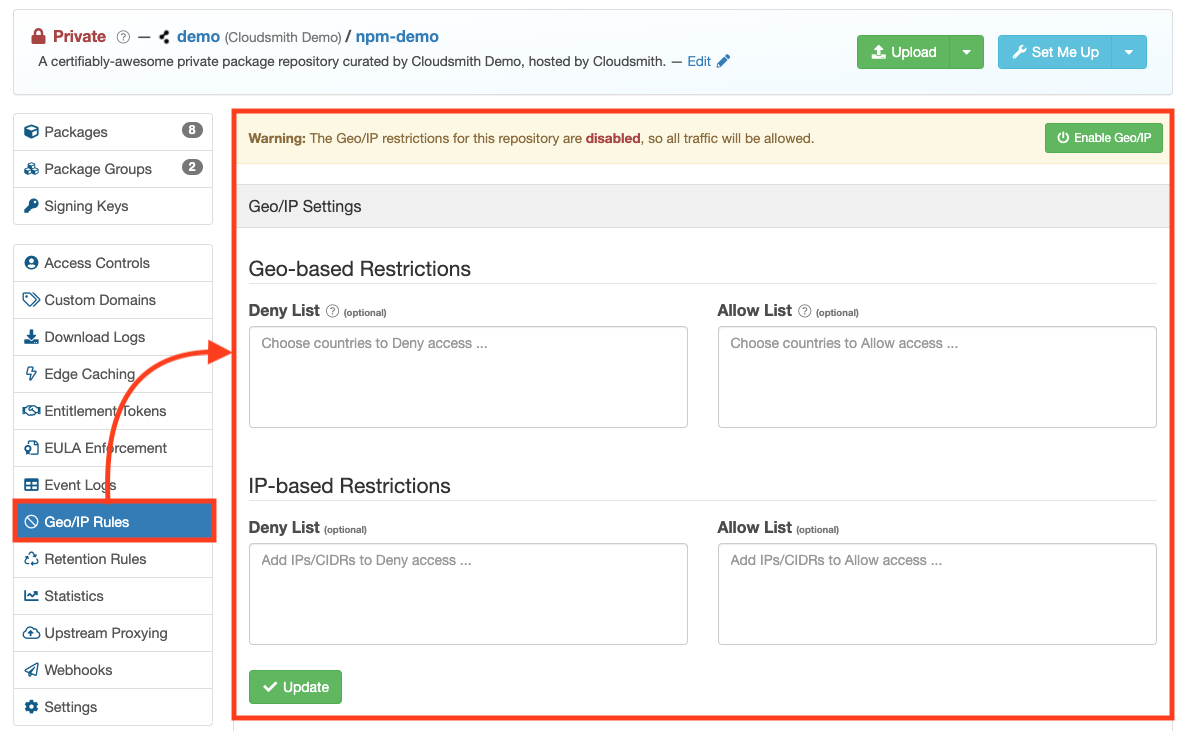This image is a detailed screenshot from a package management app or website interface. At the top, there is a light gray bar, and in the top left corner, a small lock icon is accompanied by the word "Private" in red text. To the right of this, the text reads "Demo CloudSmith Demo / NPM Demo." Below this, a descriptive tagline says, "Certifiably awesome private package repository curated by CloudSmith Demo hosted by CloudSmith." On the right side of this bar, there are two buttons: a green "Upload" button and a blue "Set Me Up" button.

Along the left-hand side of the interface, there is a vertical menu with several tabs grouped together. The first group of three tabs reads, from top to bottom, "Packages," "Package Groups," and "Signing Keys." Beneath this, a second, longer list of tabs includes various other functionalities: "Access Controls," "Custom Domains," "Download Logs," "Edge Caching," "Entitlement Tokens," "EULA Enforcement," "Event Logs," "Geo/IP Rules," "Retention Rules," "Statistics," "Upstream Proxying," "Web Hooks," and "Settings."

The "Geo/IP Rules" tab is selected, highlighted with a red outline. The main panel displays a warning at the top: "Warning: The geo IP restrictions for this repository are disabled, so all traffic will be allowed." To the right of this warning, there is a green button labeled "Enable Geo IP." Below this section, a header titled "Geo-Based Restrictions" appears, followed by options for a deny list and an allow list where countries can be specified. Users can enter countries into provided text boxes for these lists. Further down, under the header "IP-Based Restrictions," similar functionality is provided, allowing users to create deny and allow lists for specific IP addresses.